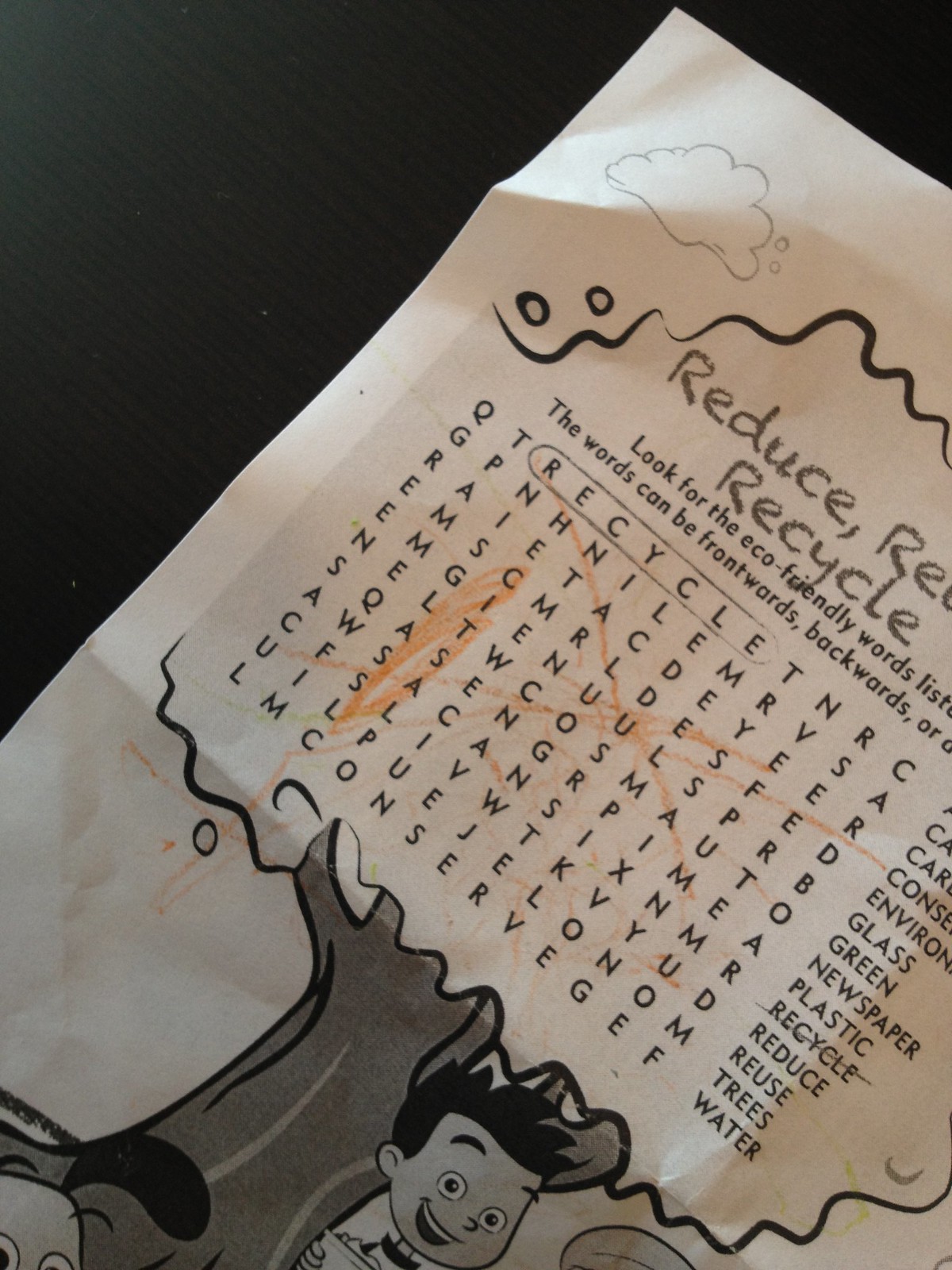The image is a close-up of the upper left portion of a page from a child's activity book, which is placed on a dark wooden surface. The background of the page is white, with black and gray illustrations and text. The page features a word search puzzle styled as the leaves of a tree, with a gray tree trunk below. The puzzle's title, "Reduce, Reuse, Recycle," prompts the child to find eco-friendly words that can be in any direction. To guide them, the word "Recycle" is circled. Additionally, the child has circled a few other words using an orange crayon. The page is slightly rotated, with a visible crease in the top left corner. A small portion of a boy’s face and a dog’s face can be seen next to the tree image. The words to find, listed on the side, include "Environment," "Glass," "Green," "Newspaper," "Plastic," "Reduce," "Reuse," and are hidden within a jumble of letters. There are also drawings of a cloud and possibly other elements partially obscured.